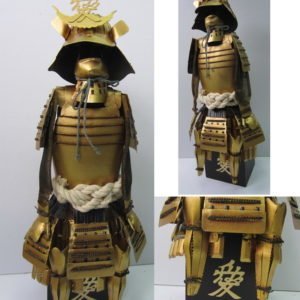The set of three photographs showcases a bronze or gold figure adorned in what appears to be samurai-inspired armor. The primary image on the left, with a gray background, highlights the full figure wearing a gold helmet that obscures most of the face except for the chin and lips. This figure is dressed in detailed armor, including a breastplate, paulders, and greaves, and is cinched at the waist with a white belt or rope. The smaller image at the top right zooms in on the upper portion of this ensemble, offering a closer view of the helmet and torso. The bottom right image, nearly square, focuses on the lower part, revealing details such as the brown section at the base with a prominent white symbol that looks like Chinese or Korean script. This intricate and multi-faceted portrayal hints at both artistic craftsmanship and cultural elements, with additional embellishments like a small necklace and possibly intricate symbols on the helmet, adding layers of historical and cultural depth.